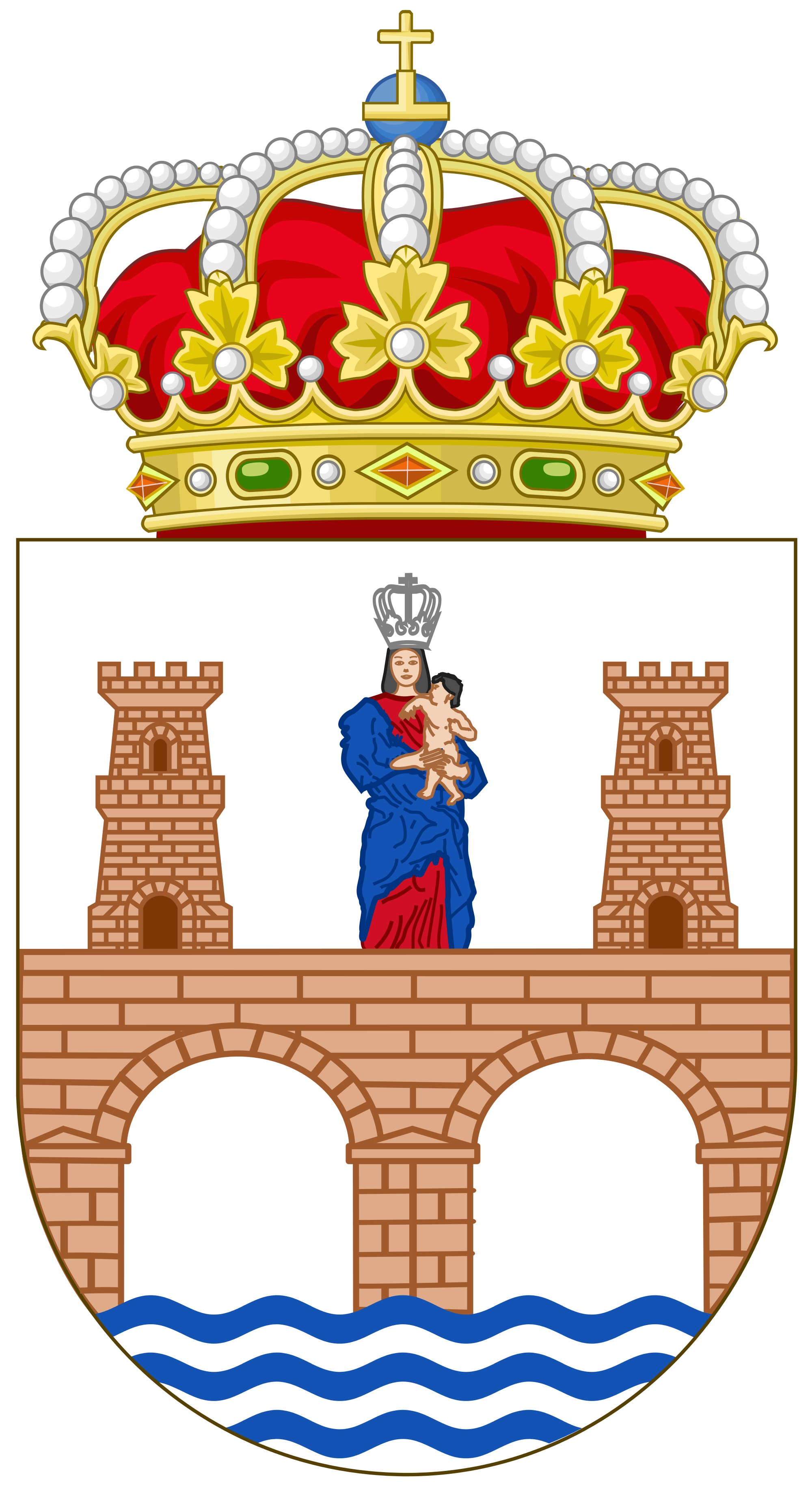The image features a detailed heraldic crest on a white background. At the top of the crest is an elaborate crown adorned with a ball and a cross. The crown itself has a design of golden bars extending upward, each decorated with white pearls. The base of the crown is richly encrusted with various gemstones, including green emeralds, white pearls, and diamonds, and finished with golden leaf patterns.

Below the crown, there is a shield-shaped emblem, flat at the top and rounded at the bottom. Inside the shield, a vivid scene unfolds: a queen wearing a silver crown, a blue robe, and a red dress, holds a naked baby. Both the queen and baby are depicted with Caucasian skin tones. The queen stands on a tan, brick bridge with two round archways beneath it. The bridge is flanked by two castle tower pillars, also made of light tan-gray bricks. At the very bottom of the shield, blue wavy lines symbolize flowing water passing through the archways of the bridge. The crown above the shield is richly detailed with gold trim and an array of red, green, and white gems, tying the entire crest together in a display of regal and historic imagery.